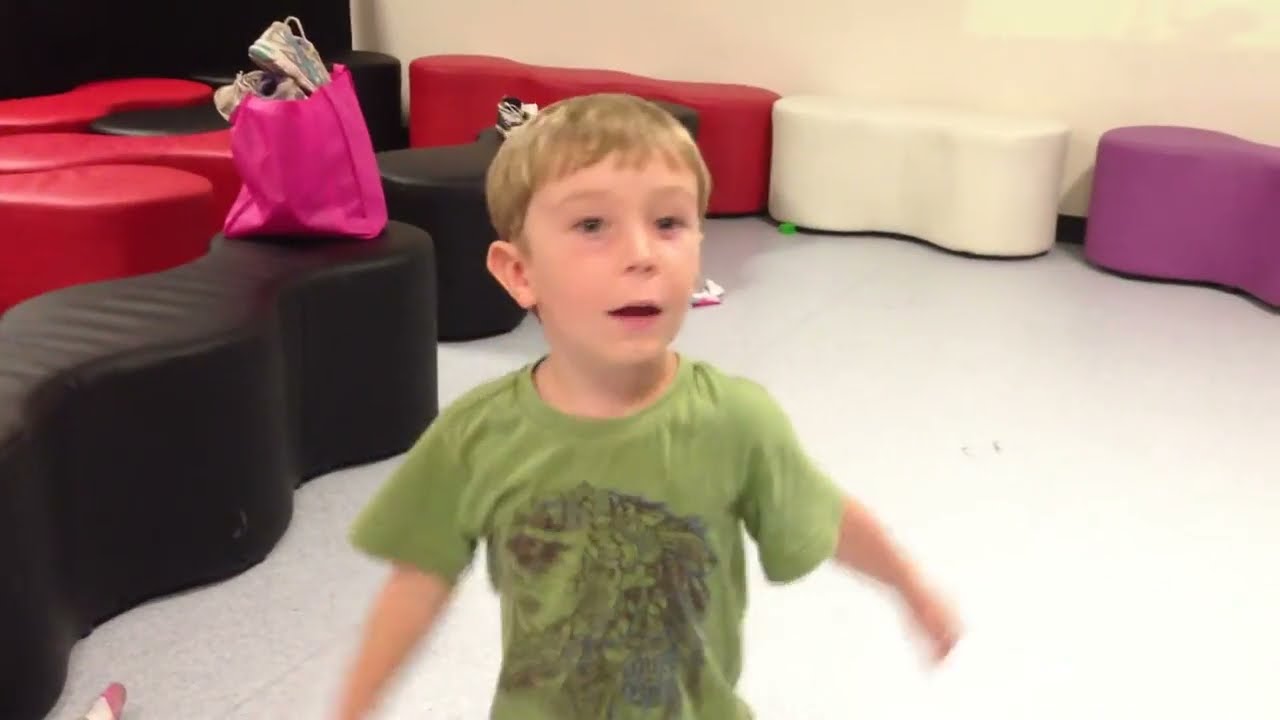In this photo, a young white boy with blonde hair is captured running around indoors on a tiled surface. He is positioned centrally, wearing a green t-shirt adorned with what appears to be a dragon design. His arms are outstretched at his sides, and he is looking directly at the camera with an intense expression, possibly caught off guard. Behind him, a collection of colorful seat cushions fills the background, featuring hues of black, red, white, purple, and tan. A bright pink bag with tennis shoes sticking out is notably placed on a black bench to the left of his shoulder. The setting is an indoor play area with a tan beige wall and a partial black wall seen to the left. Although the ground is mostly clean, a few pieces of trash and a pair of socks can be spotted scattered around. Overall, the boy seems eager to find someone to play with, adding a sense of lively anticipation to the scene.